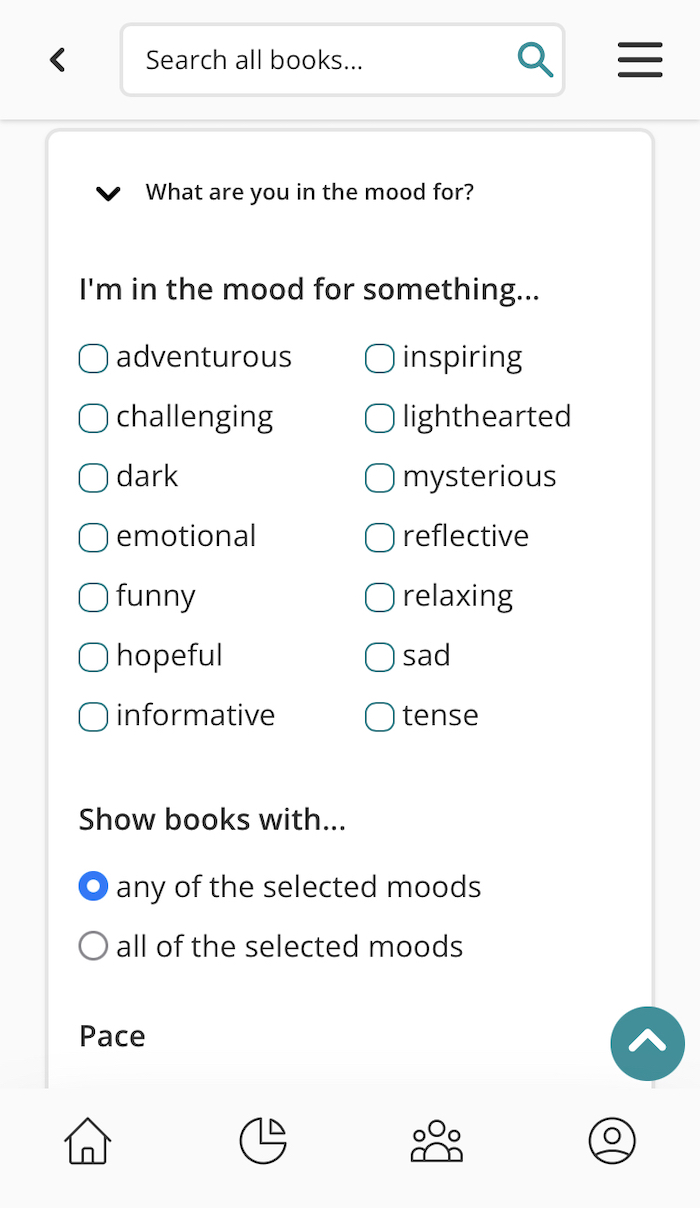### Descriptive Caption

This is a detailed screenshot from a mobile phone interface with a predominantly white background. At the top, there's a search field with the placeholder text "Search all books..." in black font. To the right end of this field is a blue magnifying glass icon, indicating the search function. Adjacent to the left of the search field is a small left-pointing arrow followed by three black horizontal lines, likely representing a menu or navigation drawer.

Below the search field, an open menu is displayed on a white background. At the top of this menu, it prompts the user with the question "What are you in the mood for?" accompanied by a small downward-pointing arrow to its left, suggesting a dropdown option. Beneath this, the text "I'm in the mood for something..." invites user interaction.

A list of mood options follows, each accompanied by a selectable circle:
- Adventurous
- Inspiring
- Challenging
- Light-hearted
- Dark
- Mysterious
- Emotional
- Reflective
- Funny
- Relaxing
- Hopeful
- Sad
- Informative
- Tense

Further down, another instruction reads "Show books with..." in black font, followed by two options for filtering:
- Any of the selected moods
- All of the selected moods

In this screenshot, "Any of the selected moods" is chosen, as indicated by the blue-filled circle to its left.